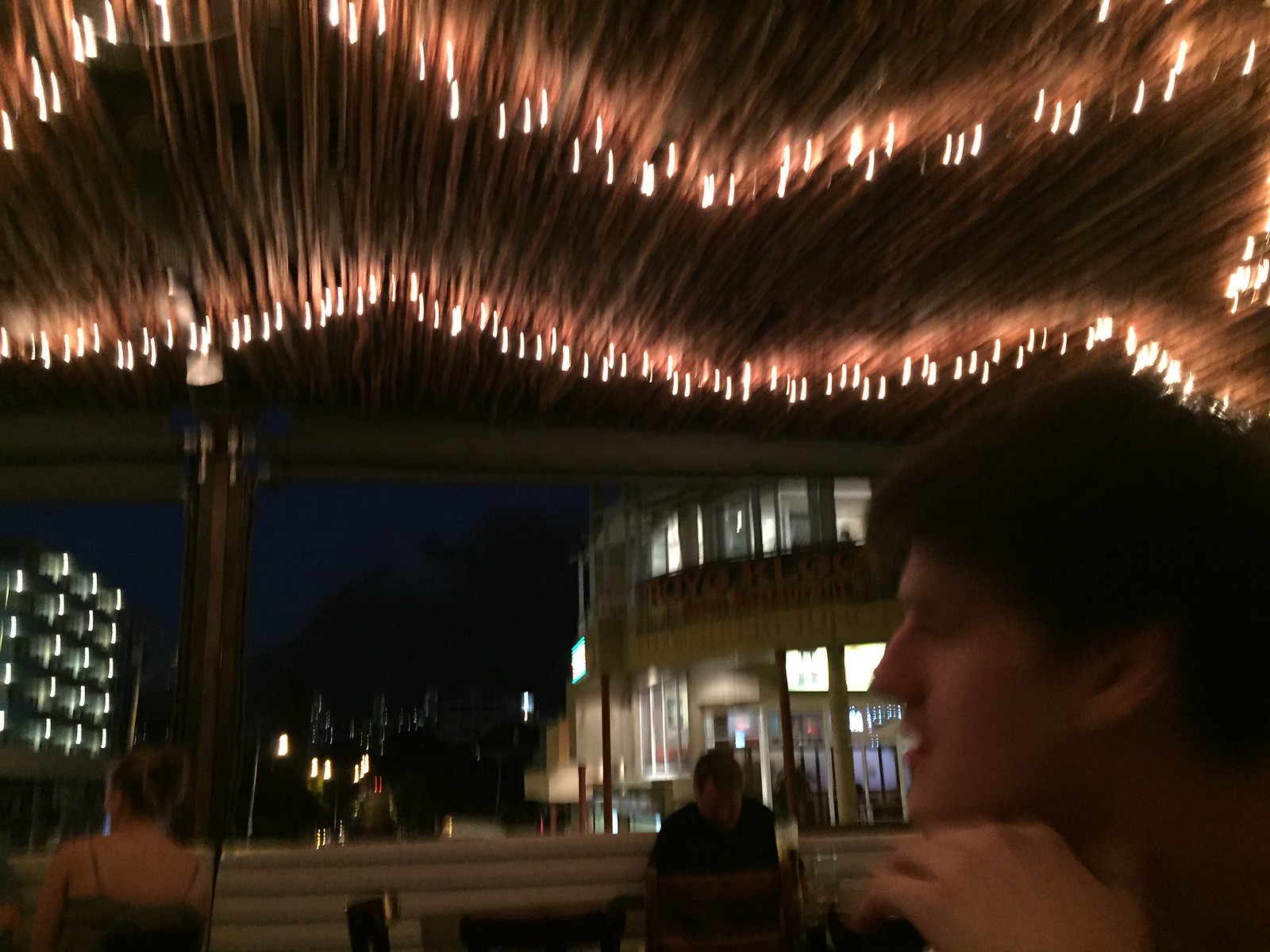This square color photograph, taken at night in a warm climate—possibly Puerto Rico or Miami—depicts the lively atmosphere of an outdoor restaurant or bar. Although the image is somewhat blurry, it captures various detailed elements and people.

In the lower right-hand corner, a white male with short brown hair sits at a table, a hand resting on his shoulder. He appears to be engaged in a conversation or perhaps in deep thought. Nearby, another man with brown hair and wearing a black t-shirt is also seated, drinking. To the left, a woman with her hair up, clad in a strappy sleeveless top, has her back to the camera.

The background reveals a brightly lit circular structure, likely a restaurant or takeaway place. Another building with lights on is visible, with a neon sign that reads "Royal Claw." The sky outside is a deep dark blue, suggesting nightfall, and some trees can be faintly seen. The ceiling of the establishment is adorned with many small lights, contributing to the overall warm and inviting ambiance. The photo, seemingly taken with a cell phone, has a slightly blurred quality, suggesting movement or an impromptu capture.